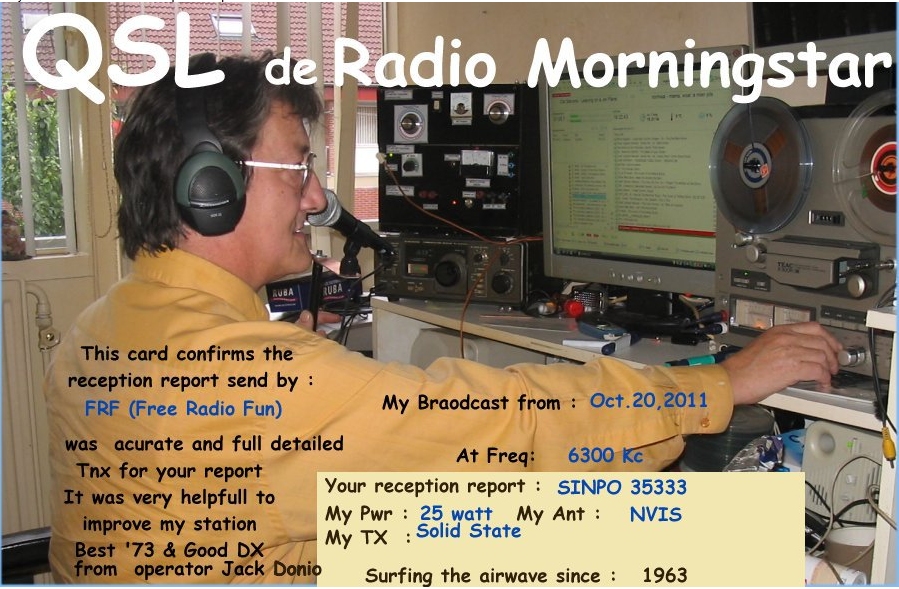The image portrays a man in a vibrant radio broadcasting studio. Wearing glasses and a light orange or yellow long-sleeve shirt, he sits comfortably in front of an array of radio equipment, with headphones over his head. He is focused, adjusting a knob on one of the devices. Prominently displayed at the top of the image is the text, "QSL to Radio Morningstar," while the bottom of the image contains detailed text, confirming the reception report from FRP Free Radio Fund. It reads, "This card confirms the reception report sent by FRP Free Radio Fund was accurate and fully detailed. TNX for your report. It was very helpful to improve my station. Best 73 and good DX from operator Jack Donio. My broadcast from October 20, 2011, at frequency 6300 KC. Your reception report SINPO35333. My power 25 W. My antenna NVIS. My TX solid state." The card also highlights "surfing the airwaves since 1963." The overall setting is well-lit, providing a clear and vibrant view of the operator and his equipment.